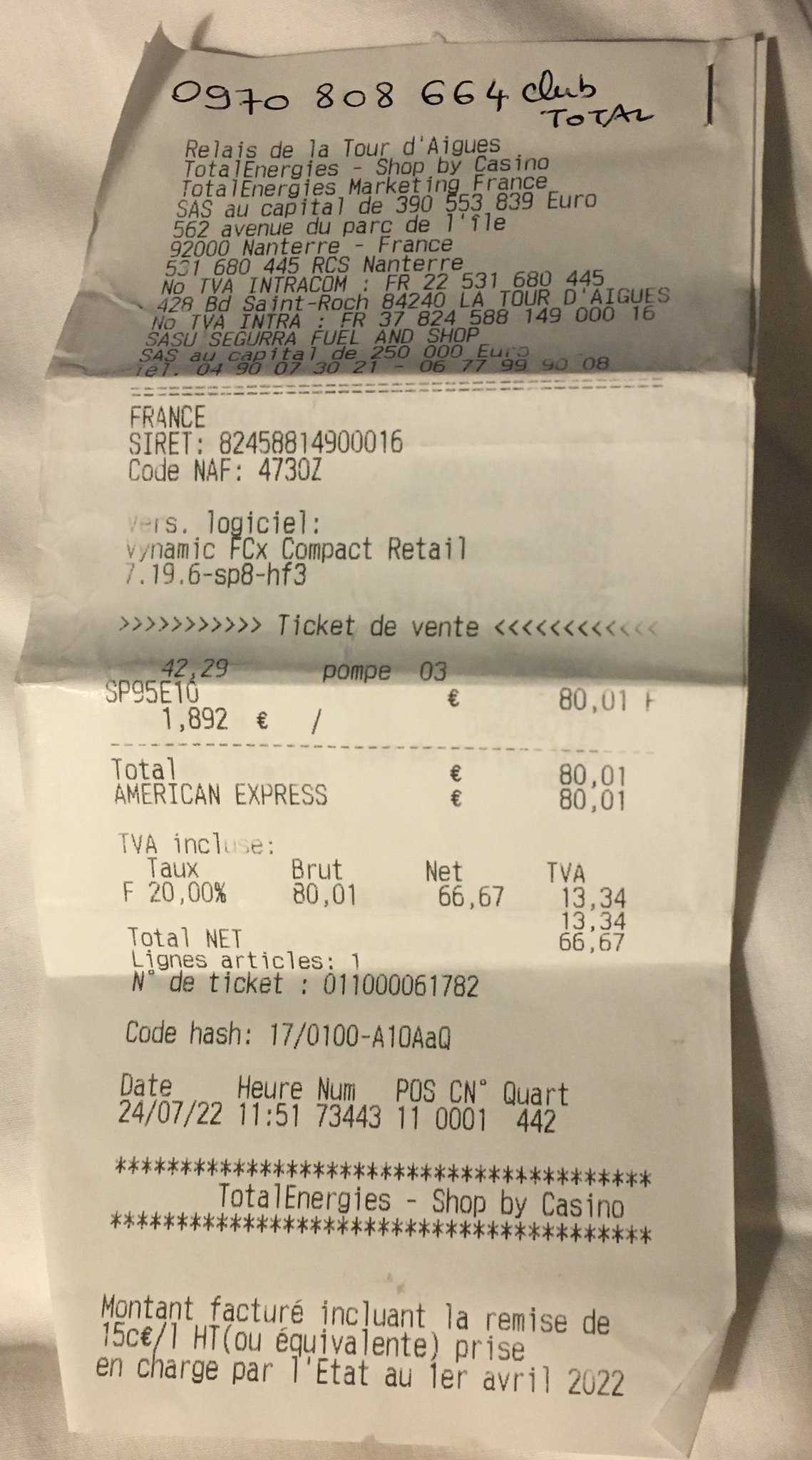The image displays a close-up of a well-folded receipt that includes both French and English text, indicating it is likely from France. At the top, there is handwritten text that reads "0970808664 Club to Car." Further down, it mentions "France" and "SIRET" followed by a sequence of numbers, suggesting it’s from a French establishment. The receipt is identified as a "Ticket de Vente," which is French for "Sales Receipt." The transaction was made with an American Express card, totaling precisely 80,001 euros. The receipt is dated July 24th, 2022, and it concludes with "Total Energies Shop by Casino," denoting the originating shop.